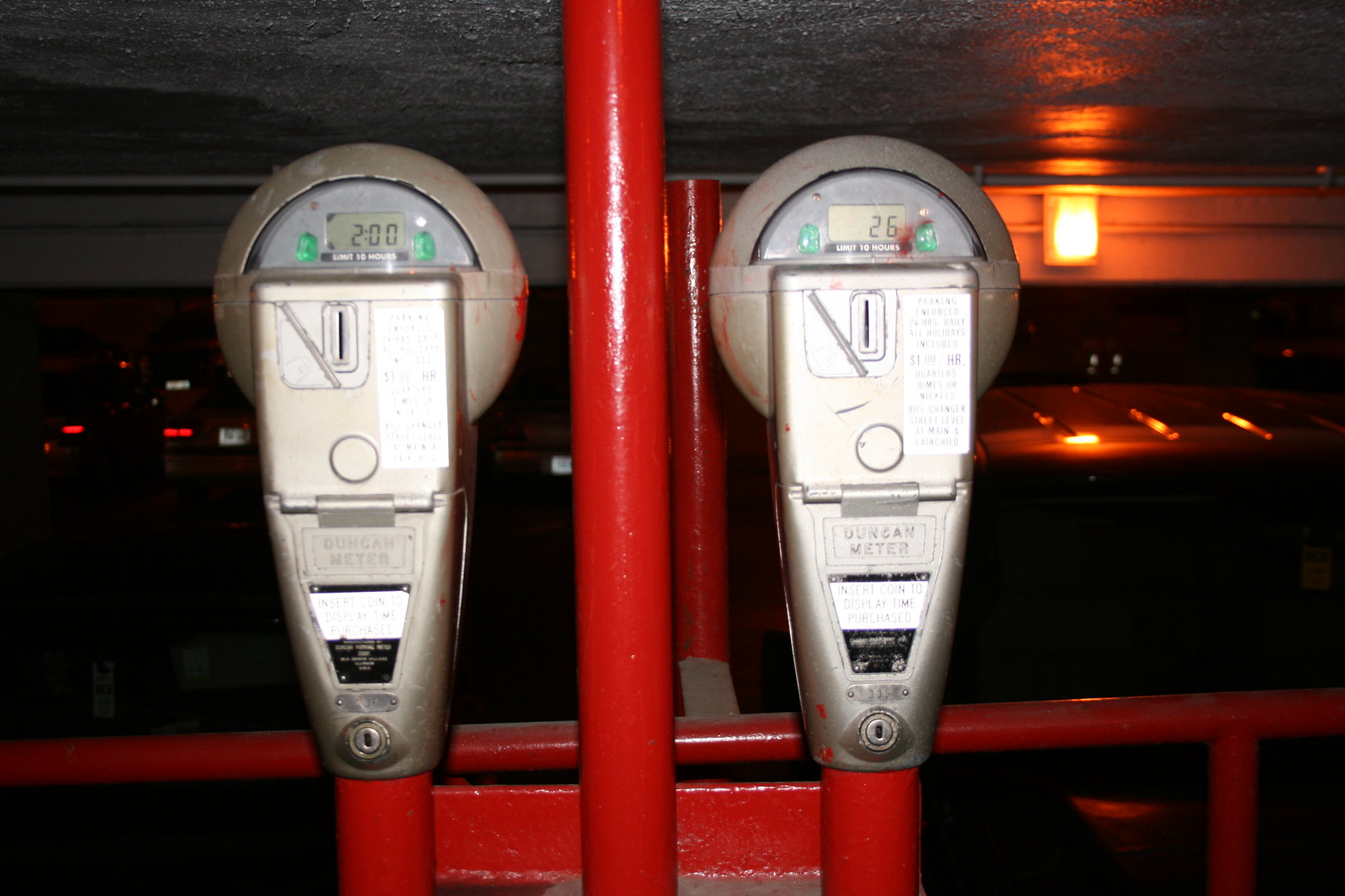This is a detailed, close-up image of two silver digital parking meters mounted side-by-side on a bright red pole structure inside a covered, well-lit parking garage. The parking meters, which are round at the top and taper down towards the pole, feature various instructions and manufacturer details inscribed in black and white medallions on the front. Both meters are currently active, with one displaying two hours remaining and the other showing 26 minutes left with their times visible from a distance on small digital screens. The red pole structure includes horizontal and vertical sections, and in the background, there are several cars parked on the opposite side of a red dividing device. The garage has a low ceiling with an orange-red light glowing, and the reflectors of the parked cars are faintly visible, further emphasizing the indoor setting.